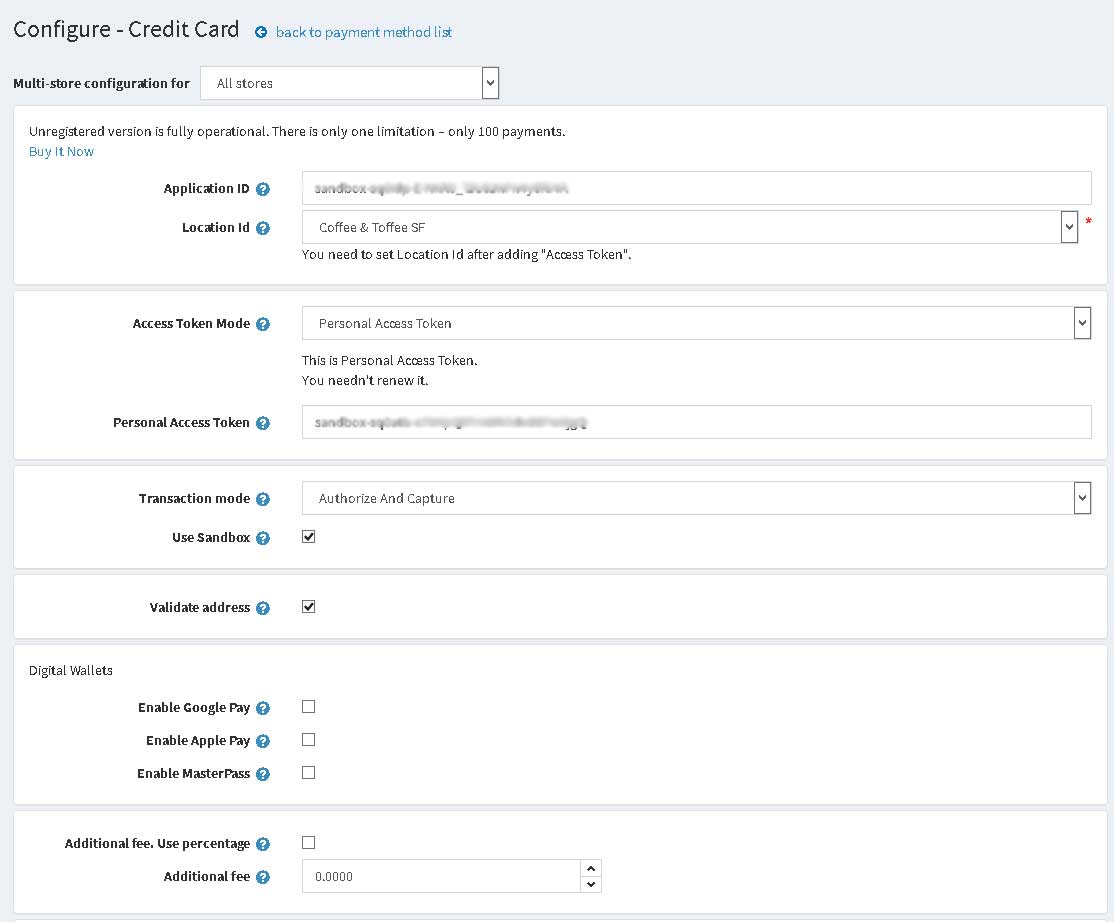A screenshot is displayed, capturing a Configure Credit Card form. The interface features approximately seven to eight form fields, which are too small to be legible. The background is grey, with multiple white text boxes spread throughout. The page appears to be a back-end configuration form likely intended for an e-commerce website. Due to the small size of the text, further details are indiscernible.